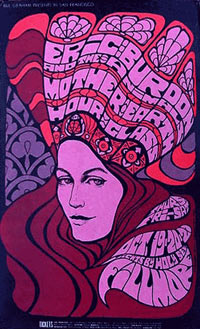This image is a portrait-oriented drawing framed with a black border, prominently featuring the face of a woman. Her facial features are highlighted with pink skin, and distinct black outlines for her eyebrows, eyes, nose, and somewhat pursed mouth, suggesting a subtle smile. The woman wears a large, intricate headdress adorned with reds, pinks, and corals, resembling the shape of peacock feathers. The headdress displays the text "Eric Burdon and the Animals," "Mother Earth," and "Hour Glass," with vibrant, psychedelic bubble letters interspersed between bright orange lines.

Her long, reddish-brown, flowing hair encircles her face and extends downwards in a swirling pattern that fills the lower part of the image. Additional text in her hair, also in distorted, bubble letters, reads "Thursday, Friday & Saturday, October 19th-21st, 2023" followed by "Fillmore," indicating that this image serves as a promotional poster for a concert event at the Fillmore venue. The overall design has an abstract, yet vibrant, 1960s psychedelic aesthetic reminiscent of artwork from that era.